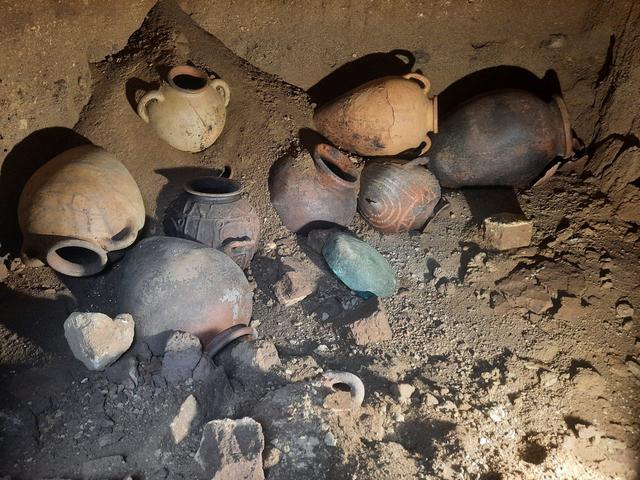The photograph captures a dimly-lit, cave-like environment, its rugged walls comprised of brown rock and dirt. Scattered across the sandy, rocky ground are various old pots, numbering around eight in total. The pots are made of clay and appear to be artifacts, each with two handles and an opening at the top. Their colors range from brown, tan, and yellow to orange, black, and bluish-gray with hints of red. The pots, some lying on their sides, are seemingly abandoned, arranged haphazardly as if tossed, contributing to the scene's neglected and disordered atmosphere. The light illuminating the image seems artificial, highlighting the pottery amidst the encompassing darkness. Also present in the image are some bricks and rocks, adding to the sense of an ancient, forgotten space filled with historical remnants.